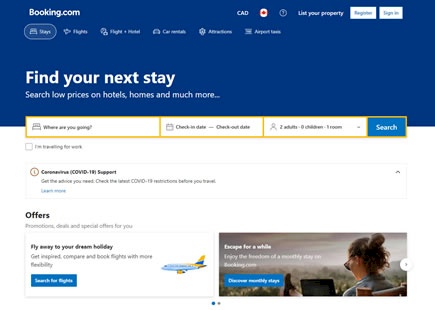A screenshot of the Booking.com homepage, featuring a distinct split layout. The top half of the page has a blue background with "Booking.com" prominently displayed in white text on the top left corner. On the top right side, there are white buttons for "Register" and "Sign in," with "List your property" and a language selection set to Canadian just to the left of those buttons. Directly beneath these are navigation tabs labeled "Stays," "Flights," "Flight + Hotel," and "Car Rentals," though some text appears blurry.

The bottom half of the page has a white background. At the top, large text encourages users to "Find your next stay" and highlights "Low prices on hotels, homes, and much more." Below this header, there are input fields and checkboxes for users to fill in their preferred accommodation details, including check-in and check-out dates, number of adults, children, and rooms. A prominent blue "Search" button enables users to submit their information.

Further down, the page mentions "Communication" and "COVID-19 support," followed by a section labeled "Offers," with green, slightly blurry text. At the very bottom, a banner advertises, "Fly away to your dream holiday," adjacent to a blue "Search for flights" button situated in the bottom left. Completing the image, there is a graphic of an airplane flying to the left on the right side of the page.